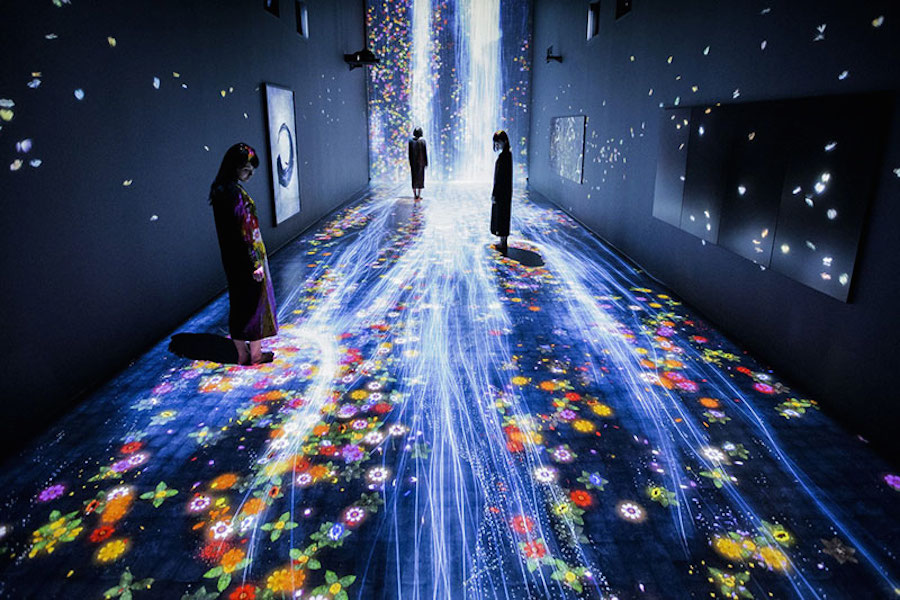The image depicts an indoor art gallery or exhibit characterized by a dark environment that effectively contrasts with various vibrant colors. The setting appears to be a hallway or corridor illuminated by numerous thin light streams and adorned with a multitude of colorful flowers projected onto a black floor. These light projections and floral designs continue seamlessly from the floor up to the wall at the end of the hallway, creating a cohesive visual experience.

On the left wall, about halfway up, there's a vertically rectangular white poster featuring an almost completely black circle. The right wall hosts a series of four vertically aligned, black rectangular panels devoid of any artwork. The predominant colors within the image include black, yellow, green, white, orange, red, light blue, light pink, and violet.

In the room, three individuals are present: a woman standing near the center left with her back to the camera, slightly facing right, wearing a purple dress; a second woman further back on the right, dressed in black and looking back towards the camera; and a third woman, also dressed in black, situated further up and looking straight ahead. This visually compelling scene captures the viewers engrossed in the intricate interplay of light, color, and floral designs, likely appreciating the immersive art installation.